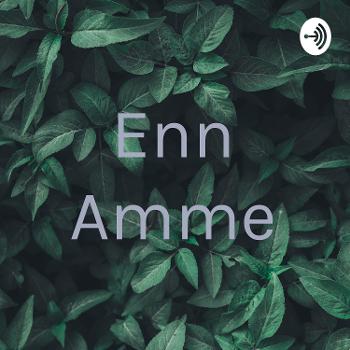The image is a square photograph featuring a background of dark green foliage with cone to oval-shaped leaves, each leaf tapering to a tip and having a vein running down its center. In the middle of the picture, text is centered both horizontally and vertically in a white or light gray font. The text on the first line reads "E N N" and on the line below, it reads "A M M E". In the upper right corner, there is a small white oval logo with a black design resembling a sideways Wi-Fi symbol: a horizontal line with three nested curved lines on the right and a small dot attached to the left. The foliage takes up the entire background, providing a lush, green setting for the text and the logo.